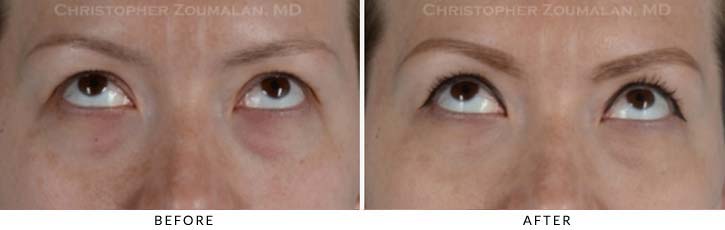This pair of side-by-side images appears to illustrate a cosmetic before-and-after transformation for a procedure conducted by Dr. Christopher Zomelan, MD. Both images focus on a Caucasian female's face, specifically from about the eyebrows to just above the end of the nose. In the before image on the left, the woman's eyebrows appear somewhat thin, and there is no noticeable eyeliner. In the after image on the right, her eyebrows are fuller and darker, and she appears to be wearing eyeliner. Additionally, her complexion looks brighter and more even. In both images, she is looking upwards, highlighting the changes around her eyes, which suggest this could be an ad for a semi-permanent or permanent makeup procedure, such as eyebrow thickening or eyeliner application.